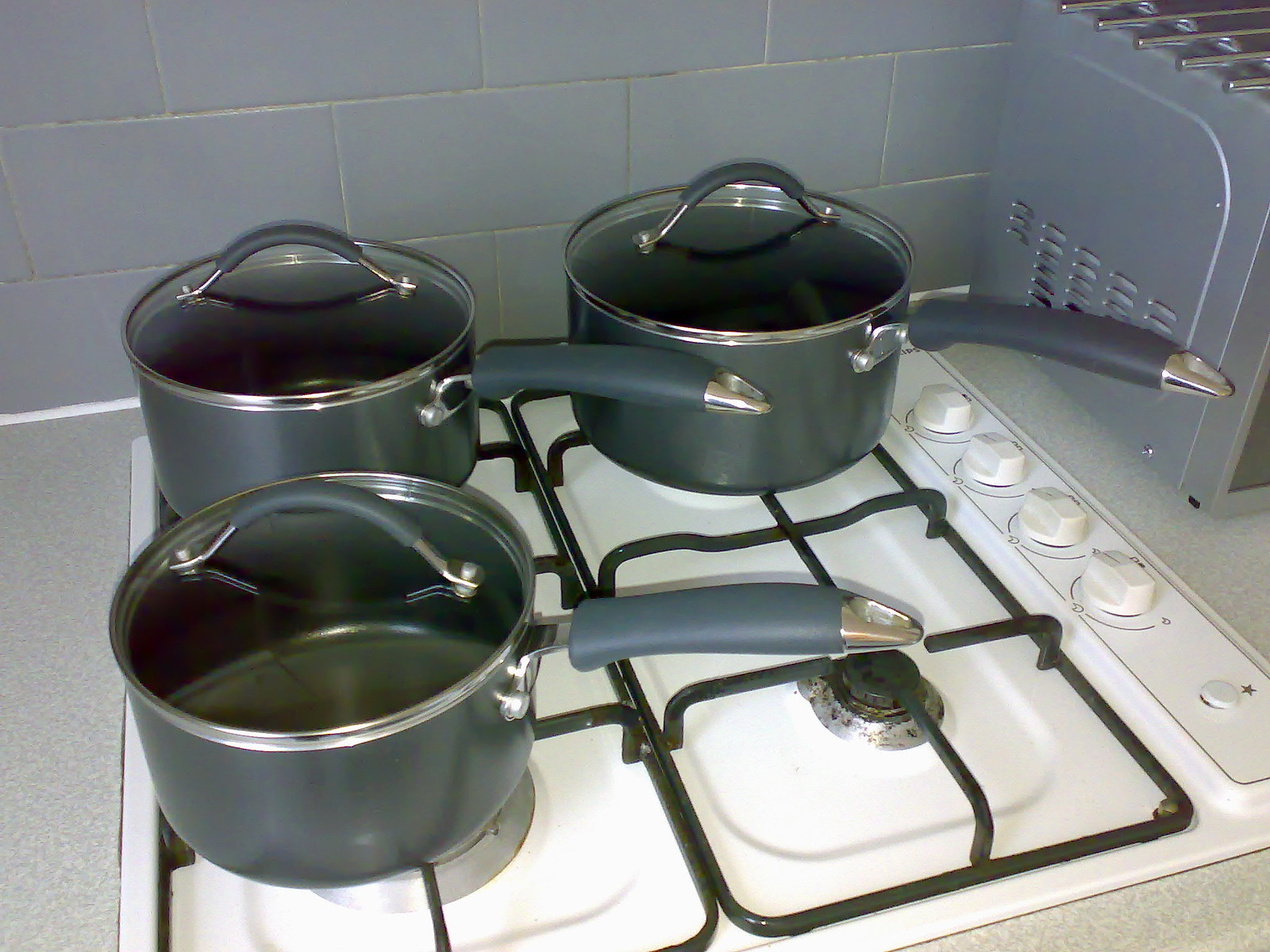This detailed photograph showcases a compact gas stove integrated into a gray, stony-looking kitchen countertop. The stove features black metal grates over a white surface and is equipped with large white dials on the right side for temperature adjustment, all currently turned off. Notably, there is a small ignition button marked by a black star. The gas stove has three dark gray saucepans with transparent lids, which reveal their empty interiors. The saucepans are positioned on the bottom left, top left, and top right burners, all with handles uniformly pointing to the bottom right. Adjacent to the stove is a grey microwave, partly visible. The kitchen background includes a subtle hint of grey tiled walls. Additionally, the handles of the saucepans are detailed with metal tips that have holes at the ends and a silver rim accentuates their design.